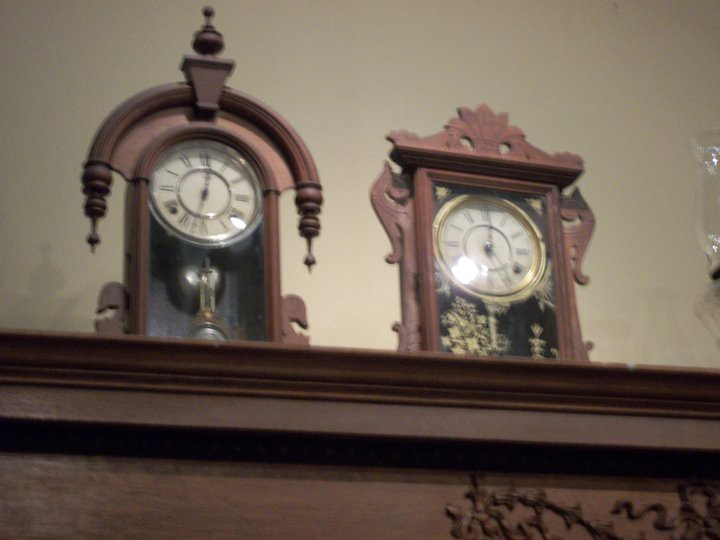The image is a meticulously detailed color photograph taken indoors, presented in landscape orientation. The focal point is on two exquisite pendulum clocks perched high on what seems to be either a high shelf or a mantelpiece, inferred from the upward-tilting camera angle. Dominating the lower horizontal edge of the image is a subtly embossed wooden ledge, featuring intricate detailing that suggests it could belong to an ornate cabinet or the front of a mantelpiece.

Each clock, crafted from finely lathed wood, boasts ornate designs and features a glass or plastic front through which parts of the pendulum are visible. The left clock reveals a glimpse of the circular top of its pendulum, while the right clock shows only its pendulum arm. Both clocks display traditional analog faces. Illuminating the scene, light from either an indoor source or the camera's flash reflects brightly off the clock faces, adding a dynamic interplay of light to the photograph.